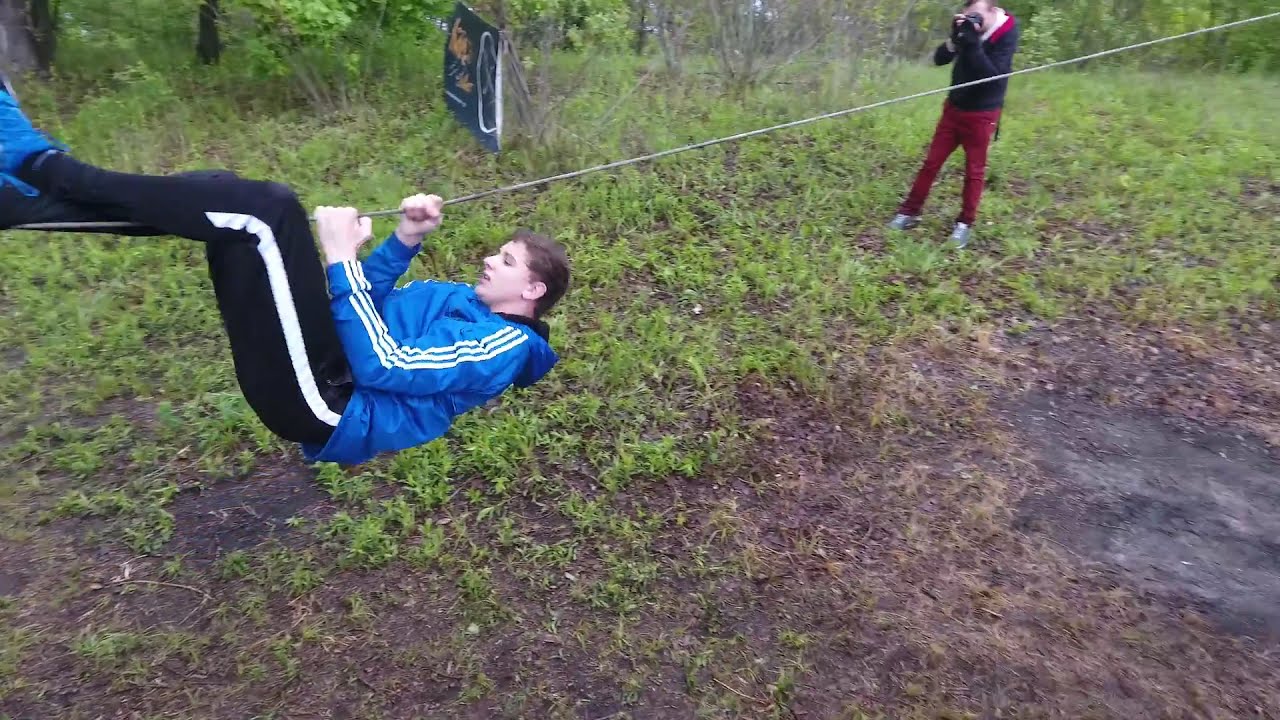In this photograph, a young Caucasian man with brown hair is seen climbing along a wire, suspended roughly three feet above the muddy, grassy ground. The young man is dressed in a royal blue, waterproof track jacket adorned with white stripes down the sleeves, and he pairs this with black pants that feature a white vertical stripe along the leg. His blue and black sneakers hint at an active and sporty nature. Utilizing both his hands and legs, the man exhibits significant upper body strength as he hangs below the wire, facing to the right with his body extended horizontally.

The setting appears to be a natural outdoor environment, possibly a forest or jungle, as evidenced by the surrounding trees and patches of green grass intermingling with the muddy ground. On the right-hand side of the image, a second Caucasian man is captured photographing the climber. This photographer dons a black top with red pants and holds a large black camera up to his eye, intent on capturing the determined expression of the climber. A small, partially obscured black sign with yellow and white images is also visible in the background, adding an element of curiosity to the scene. The overall atmosphere reflects an adventurous, physically challenging moment set amidst the calmness of nature.